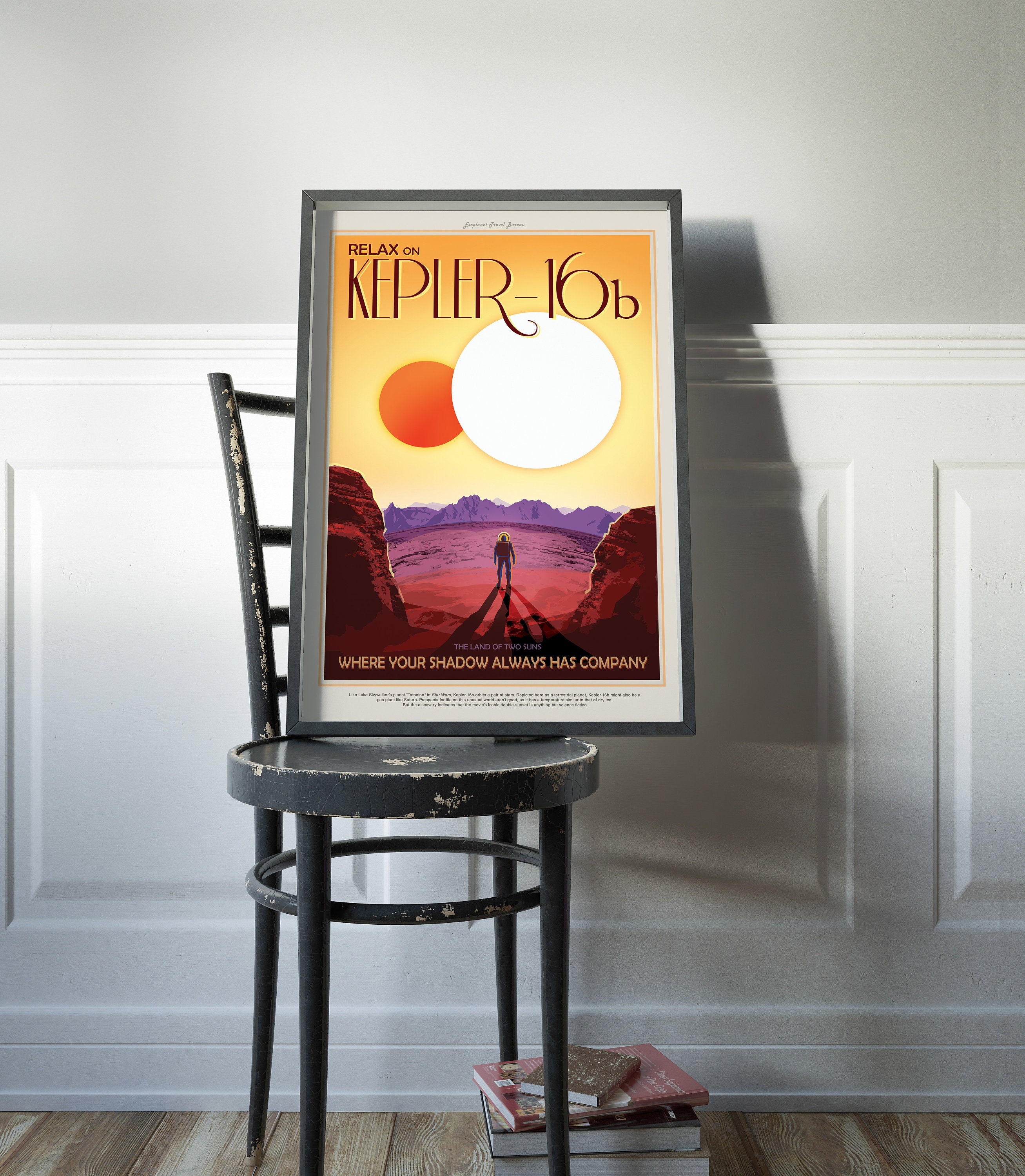The image depicts a room featuring a worn gray chair placed against a white wall that transitions to a gray wall above a wooden floor. A few closed books are stacked on the floor near the chair. On the chair is a framed poster with a gray frame, featuring the text "Relax on Kepler-16B" at the top. The poster showcases an abstract celestial scene on a yellow background: a large white circle representing a sun, and a smaller orange circle, perhaps a secondary star. Below this, a figure, presumed to be a man wearing a hat, stands on a red-hued ground with reddish stones nearby. The text at the bottom of the poster reads "Where your shadow always has company," with an illustration of the man's shadow clearly visible.